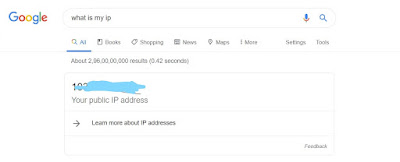In the image, a Google search result is displayed for the query "What is my IP?" At the top, beneath the search bar, there are navigation options such as AI, Books, Shopping, News, Maps, More, Settings, and Tools. The search query yielded approximately 2 million results in about 0.42 seconds. The screen shows a large block of blue paint scribbled over the actual IP address, with the text "Your public IP address" indicating its location. Below this, there are links to "Learn more about IP addresses" and "Feedback." The Google logo is visible next to the search bar, and there is also an icon for voice search.